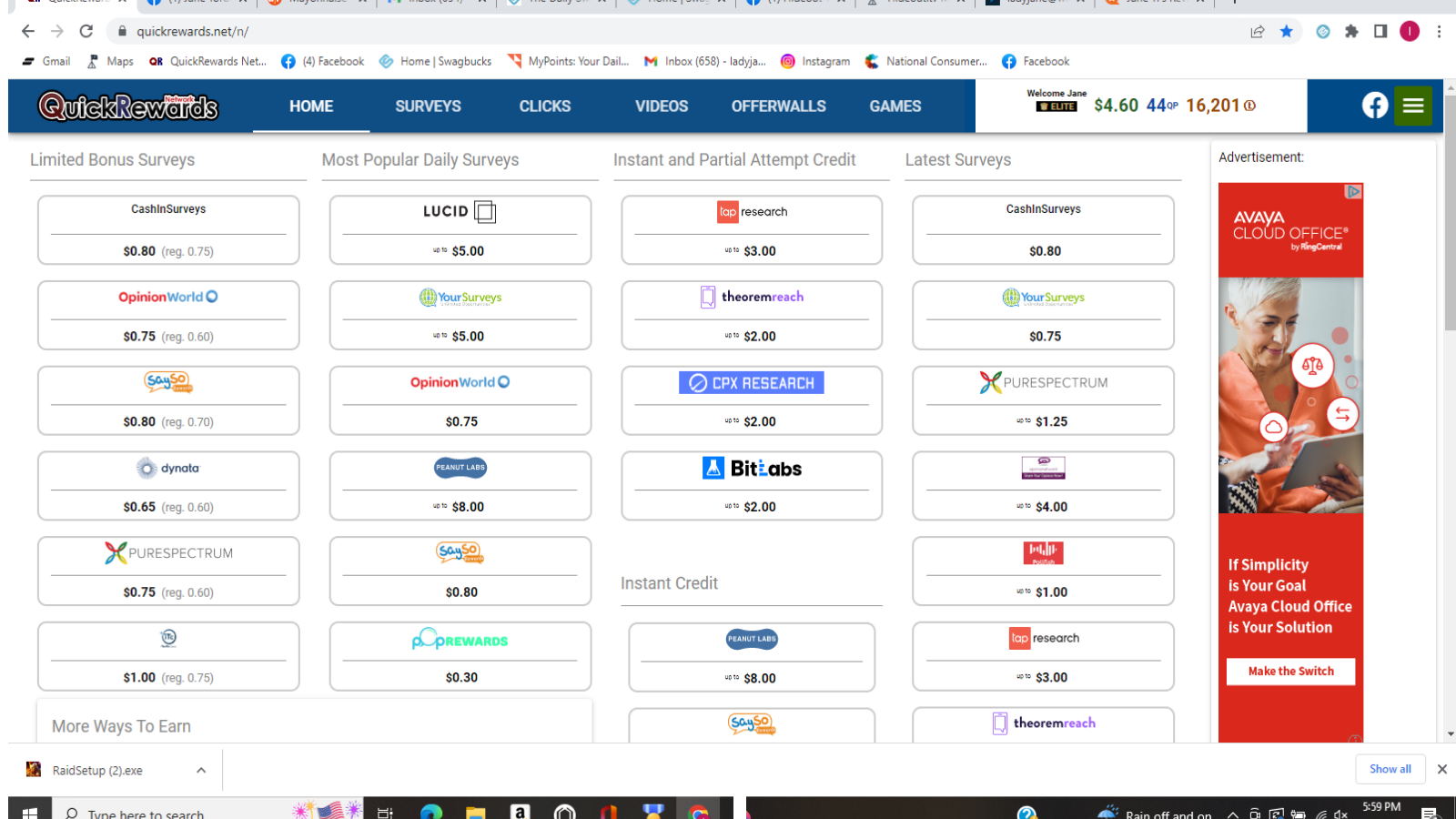The screenshot displays a survey rewards website, captured in a rectangular format with longer top and bottom sides. At the very top, the browser interface is visible with multiple open tabs, most of which are cut off at the edges of the screenshot. The URL bar, displayed as a long box with curved ends, contains the text "quickrewards.net/n/".

Below the browser interface, a blue banner spans the top of the webpage. On the far left, the banner features the site name "Quick Rewards" in black text. The banner also includes navigation options in white text: "Home," "Surveys," "Clicks," "Videos," "Offer Walls," and "Games." 

Towards the right side of the banner, there is an embedded white rectangle. It welcomes the user with the text "Welcome Jane" and displays several stats: "$4.60" in green text, "44 QP" in blue text, and "16,201" in red text.